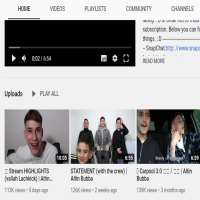The image features a gray background with a navigation bar at the top that includes clickable options for "Home," "Videos," "Playlists," "Community," and "Channels." Below the navigation bar, there is a video player displaying a paused video at a timestamp of 2 minutes and 2 seconds out of a total duration of 6 minutes and 54 seconds. The progress bar does not appear to align with the 2:02 timestamp, suggesting it may be stuck or frozen. To the right of the video player, there is small, indistinct text accompanied by a blue hyperlink that is too blurry to read, followed by a light gray horizontal line.

Beneath this section, there is the word "Upload" followed by a right-pointing triangular play icon and the text "Play All." Further down, there are three video thumbnails arranged horizontally. Each thumbnail features a black box in the bottom right corner displaying the video's duration, small and blurry text below the image, and additional information about the number of views and the time since it was posted. The leftmost thumbnail depicts a man in a white shirt, smiling and looking directly at the camera.